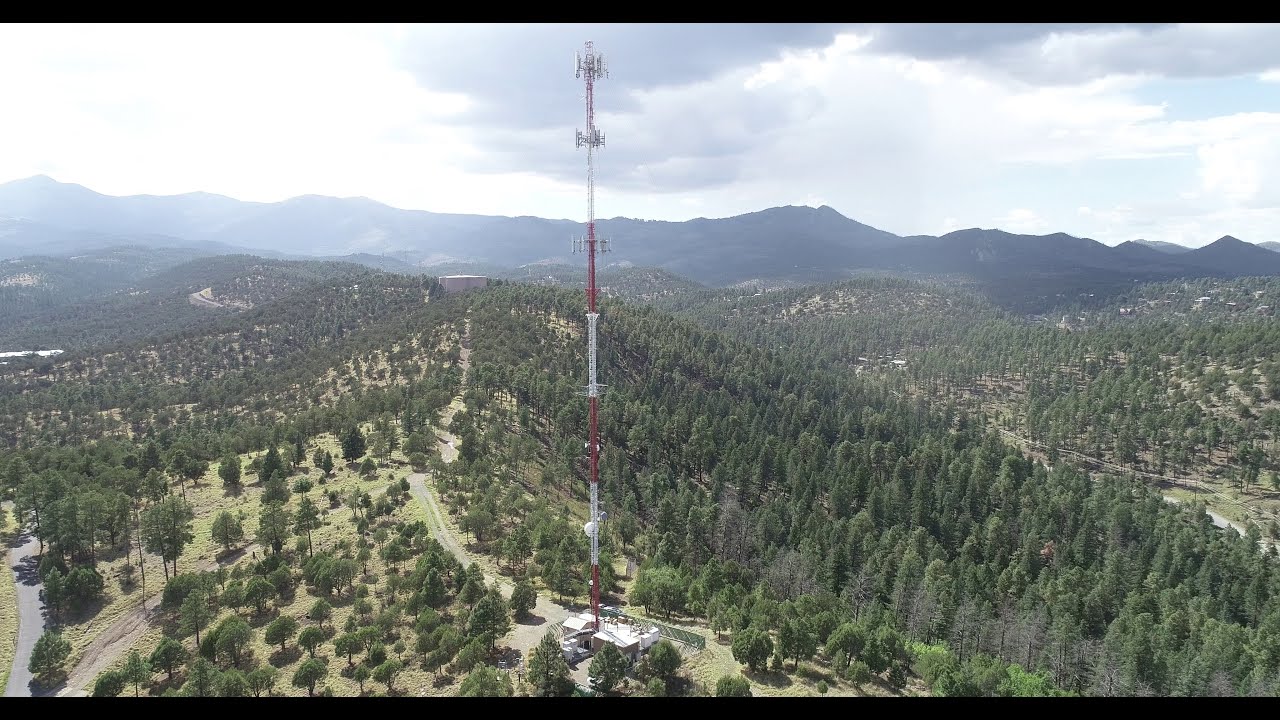In the foreground of this detailed and expansive aerial view, a prominently tall radio tower stands out against the natural backdrop. The tower is segmented alternately in dense sections of red and white paint. The base of the structure appears to be supported by a large white platform, and it houses various fixtures such as radio or cellular equipment. The middle and top sections of the tower also feature additional equipment, likely for broadcasting or communication purposes.

Situated on a hill amidst a densely forested landscape, the hill features thinly sparsely distributed trees on the left, while a thick forest stretches out to the right. A small pass or road cuts through the hillside leading up to the tower, which includes a cluster of buildings at its base—some appearing to be large, single-story equipment sheds and others, possibly, a two-story building. A fence partially encloses the area to the right.

In the background, more mountain ridges rise dramatically. These rocky formations have sharp points and are interspersed with dark shadows cast by the overcast clouds. The sky above is filled with thick, varied clouds, some darkening at the bottom, adding to the rugged and untamed beauty of this rural scene.